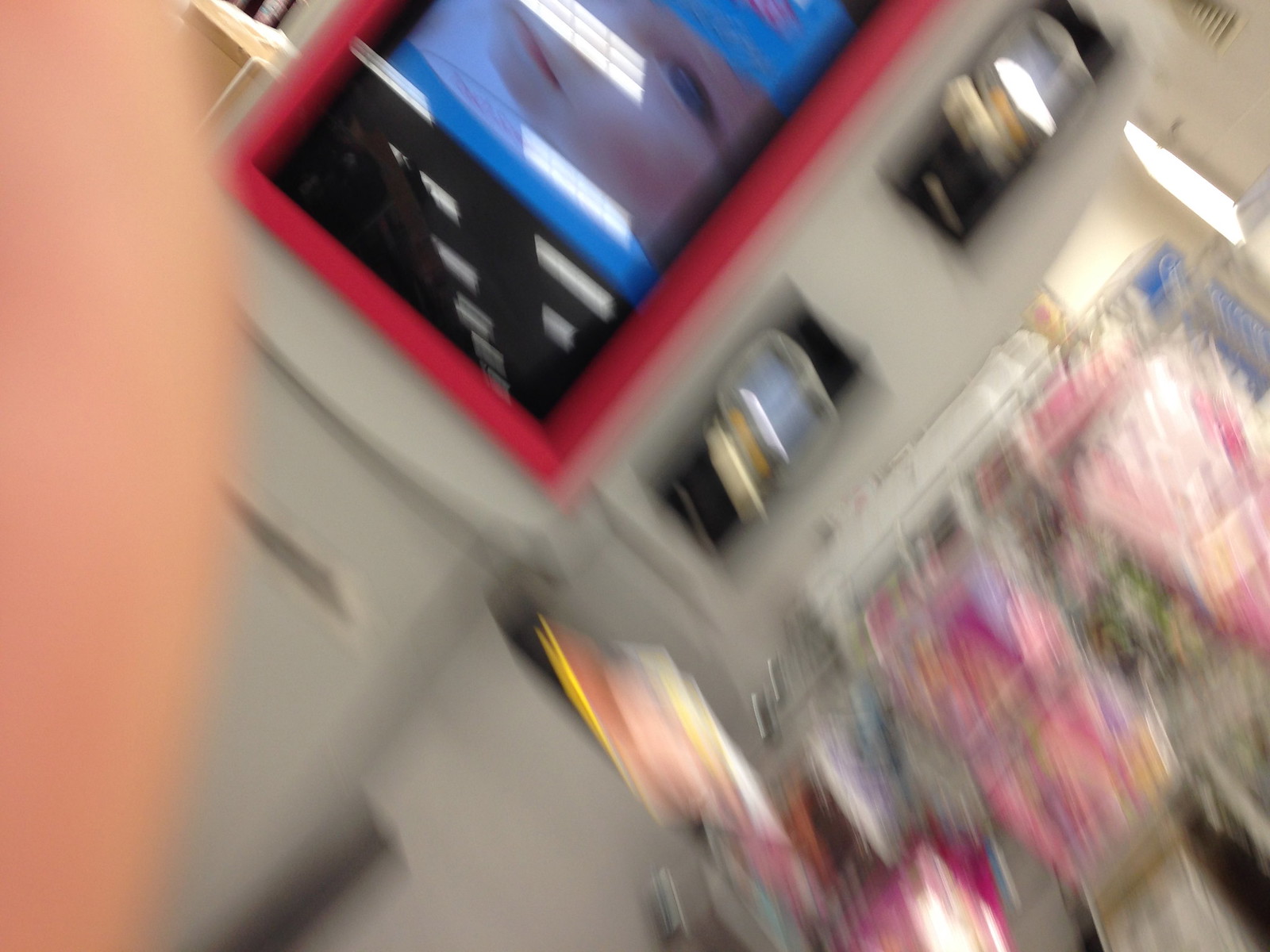A blurred photograph inadvertently taken inside a store, likely snapped by mistake. The camera seems to have been positioned around hip height, and a finger partially obscures the lens, suggesting the photo was accidentally taken while pulling the phone from a pocket. Visible in the image is a screen displaying a baby, along with reflections of store lighting on the screen. Surrounding the screen, a display rack holds pink merchandise, and the overall color palette includes gray hues from the store's walls and flooring.